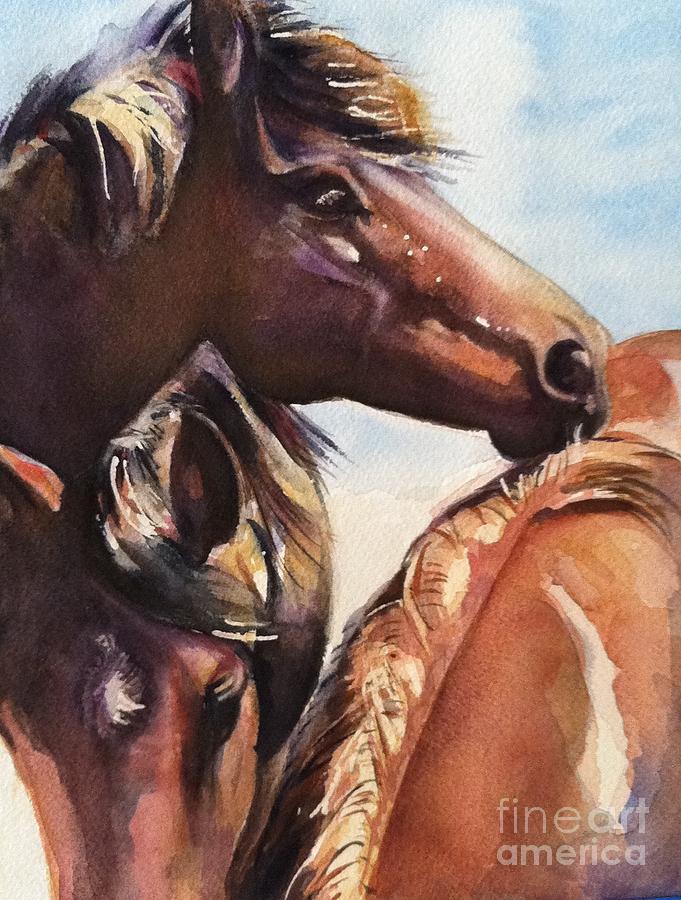The image is a vertically oriented, rectangular watercolor painting depicting three brown horses with some white markings. At the top of the image, a horse's head is shown in profile, facing to the right, with portions of its mane falling over its neck and cascading across its chest. This horse has white spots on the top of its nose and mouth area. Immediately below, another horse's head faces the viewer, slightly lowered, revealing a white patch in the center of its forehead. The two visible horses both have chocolate-brown coats and dark manes with hints of tan. Additionally, part of a third horse's body and neck can be seen along the right side and bottom right corner of the image. The background features blue sky and clouds. In the bottom right corner, the text "Fine Art America" is visible.